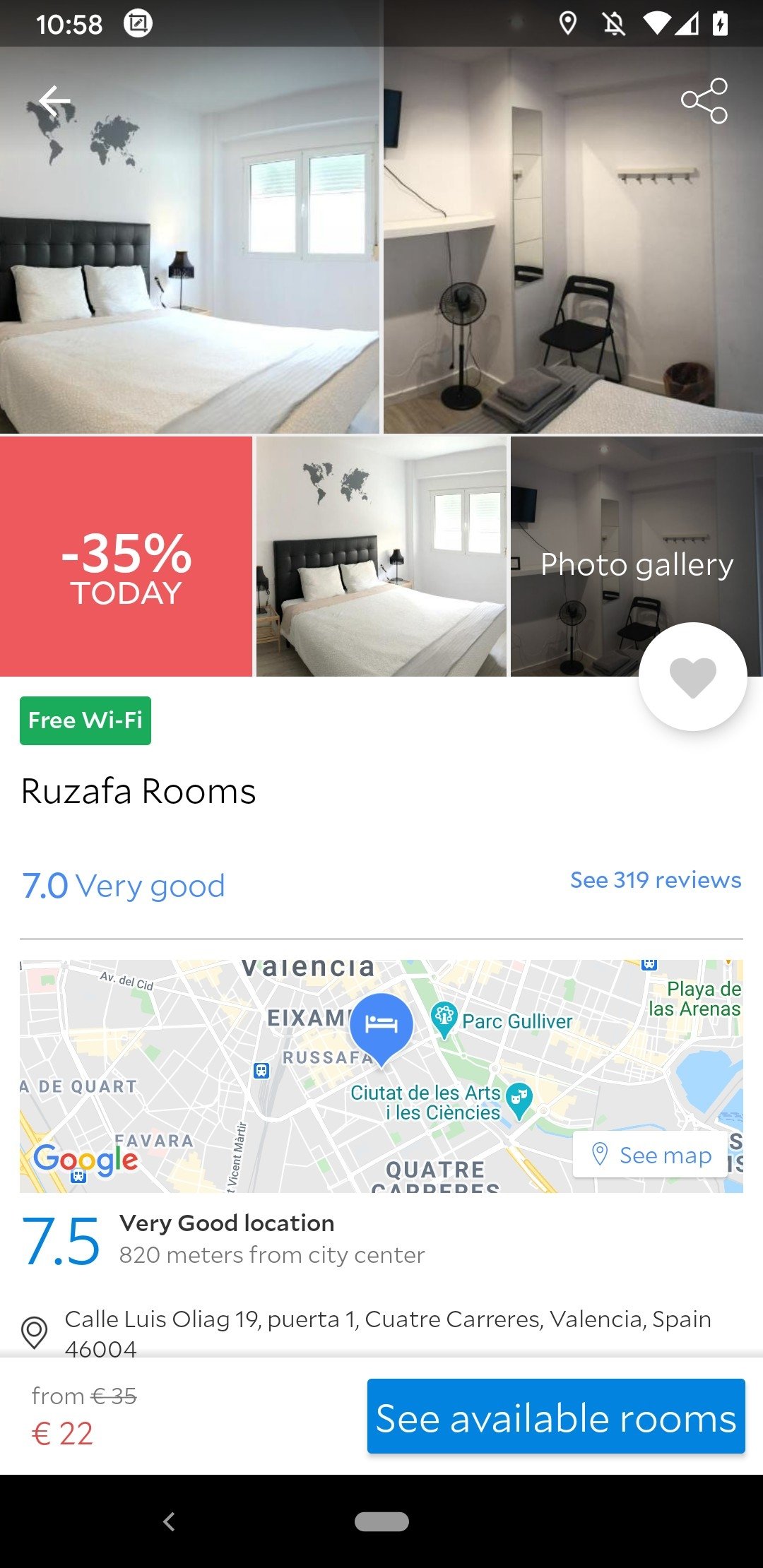The vertically rectangular image is a screenshot from a cell phone, showcasing a detailed informational page for "Ruzafa Rooms." The header includes a narrow black banner displaying the current time, "10:58," on the left, and a series of icons on the right indicating location services, an inactive alarm, Wi-Fi, signal strength, and battery life.

Below the banner are four thumbnail images arranged in two rows. The top row features two interior photos of the accommodation. Among the bottom row, the left image stands out with a red background and a "Minus 35% Today" text highlighting a discount. The center image is a smaller version of the top-left interior photo, and the rightmost image provides a clickable link to a photo gallery for more pictures.

Highlighted in green text below the images is the phrase "Free Wi-Fi," followed by the name "Ruzafa Rooms," which has a rating of "7.0, Very Good" based on "319 reviews." Next, there is a horizontally rectangular map with a pinpoint indicating the exact location.

Further details reveal a rating of "7.5, Very Good" for the location, which is "820 meters from the city center." The address is provided as "Cuatre Carreres, Valencia, Spain."

At the bottom right of the page is a prominent blue button labeled "See Available Rooms," inviting users to check room availability.